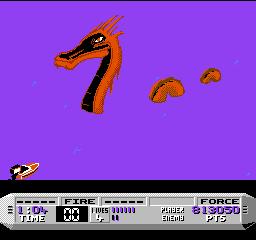This image features a vivid screenshot from a video game, set against a bright purple background. Dominating the scene is a striking orange and black dragon-like sea creature, reminiscent of a serpent, with distinct segments of its neck and tail visible as it arches out of the water. In the bottom left corner, a small boat, depicted in orange, white, and black, appears to be navigating towards the creature. At the bottom of the image, a grey HUD (Heads-Up Display) provides various game statistics: on the left, a black box contains white lettering '00', indicative of time or points remaining; nearby, text elements read 'Fire', 'Force', '1-04', and '813050' alongside 'PTS', likely denoting points scored; additional numerical details and descriptors such as 'player' and 'enemy' are also displayed, framed by black and grey outlines. The intricate details and vibrant colors suggest an intense and immersive gaming experience.